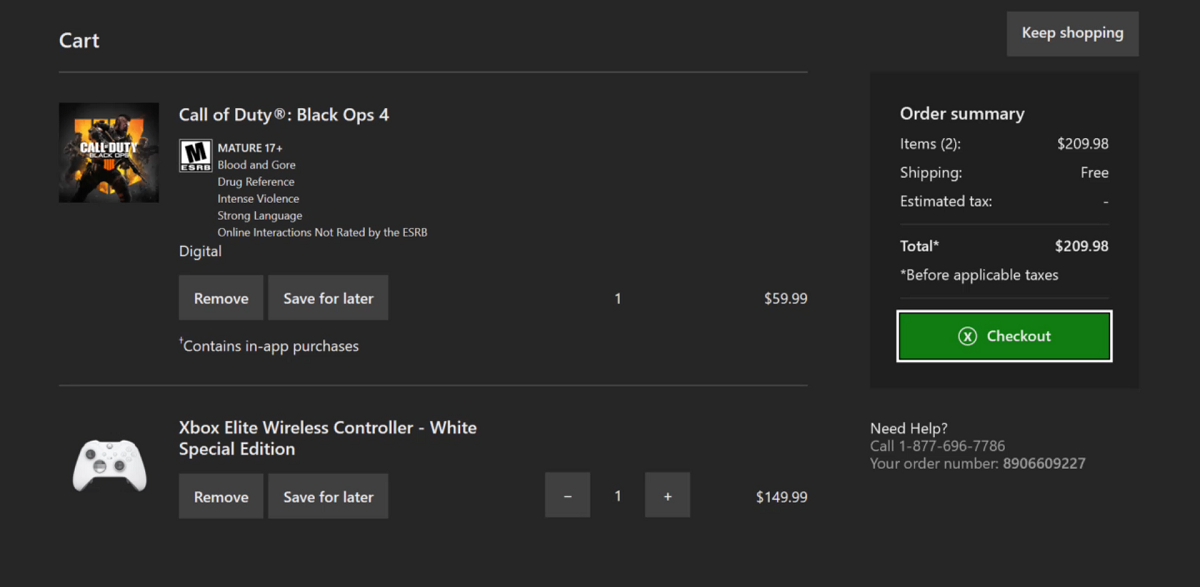This screenshot depicts an online shopping cart interface with a black background and detailed elements arranged to facilitate the user’s shopping experience.

In the top left corner, the word "Cart" is prominently displayed in white text. The interface’s layout is approximately twice as wide as it is tall. On the top right, just an inch from the edge, a lighter gray tab with white text reads "Keep shopping." Beneath the "Cart" heading, a horizontal line spans about two-thirds of the screen's width. 

Within this section, starting from the left, there is an image associated with the video game **Call of Duty: Black Ops 4**. The cover features a man with a mohawk and a beard, holding a gun pointed downward. Superimposed on this image are the game's title "Call of Duty" and "Black Ops 4" in white text along with an "R" symbol for trademark. Below this image sits the "Mature 17+" rating logo. Further to the right of this, there are options available in gray tabs labeled "Remove" and "Save for Later.” The game is marked as digital content under "contains in-app purchases" visible beneath these tabs. This item is priced at $59.99 on the far right, next to a quantity indicator of '1'.

Separated by another horizontal line, the next item featured is an **Xbox Elite Wireless Controller - White (Special Edition)**. The picture of the controller is positioned on the left. To the right, the item's title is presented, with additional details like "Special Edition." Similar to the game listing, gray tabs here also offer "Remove" and "Save for Later" options. This controller is priced at $149.99, with a quantity of '1'.

To the right, next to the "Keep shopping" tab, there is a rectangular section outlining the order summary. This includes information on the number of items, cost breakdown, shipping, estimated tax, and the total amount before applicable taxes. A striking green button featuring a white-bordered circle with a white "X" and the word "Checkout" in white text sits at the bottom of this summary.

Below the order summary rectangle and extending into the gray background, there is a "Need help?" section accompanied by a customer service phone number and your order number, providing easily accessible support.

Overall, this detailed and organized layout ensures a seamless shopping experience.